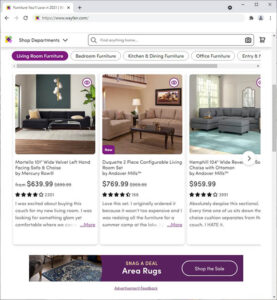This image appears to be a small screenshot of a furniture retail website, which primarily showcases an array of couches available for purchase. There are three distinct image thumbnails, each featuring a different couch model. Accompanying these images are price tags: the first couch is labeled at $639, the second at approximately $769, and the third at about $959. Directly beneath each couch image is a brief description providing general information about the respective item. Positioned at the top of the webpage is a search bar, enabling users to look for additional items not displayed on the current page. The website's platform and specific site name are not identifiable from this image. However, it is clear that the site's primary function is to facilitate the sale of furniture.